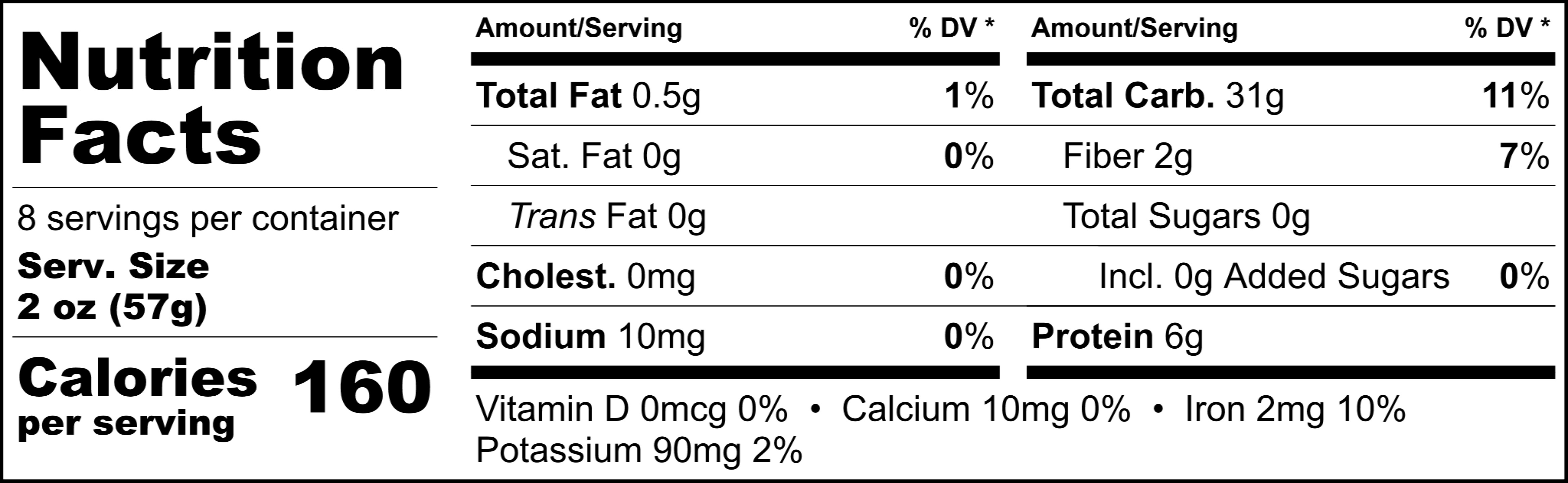This image displays a monochromatic, rectangular nutrition label in a standardized format. The label indicates that the product contains eight servings per container, with each serving size being two ounces. Each serving provides 160 calories. Notably, the label shows negligible amounts of fat and cholesterol. It also includes minimal dietary fiber at two grams and lacks significant vitamins, with only 10% of the daily value for iron and no vitamin D or calcium. The product contains six grams of protein and 31 grams of carbohydrates per serving. Given the generalized and simplistic design, the specific nature of the product remains indiscernible.